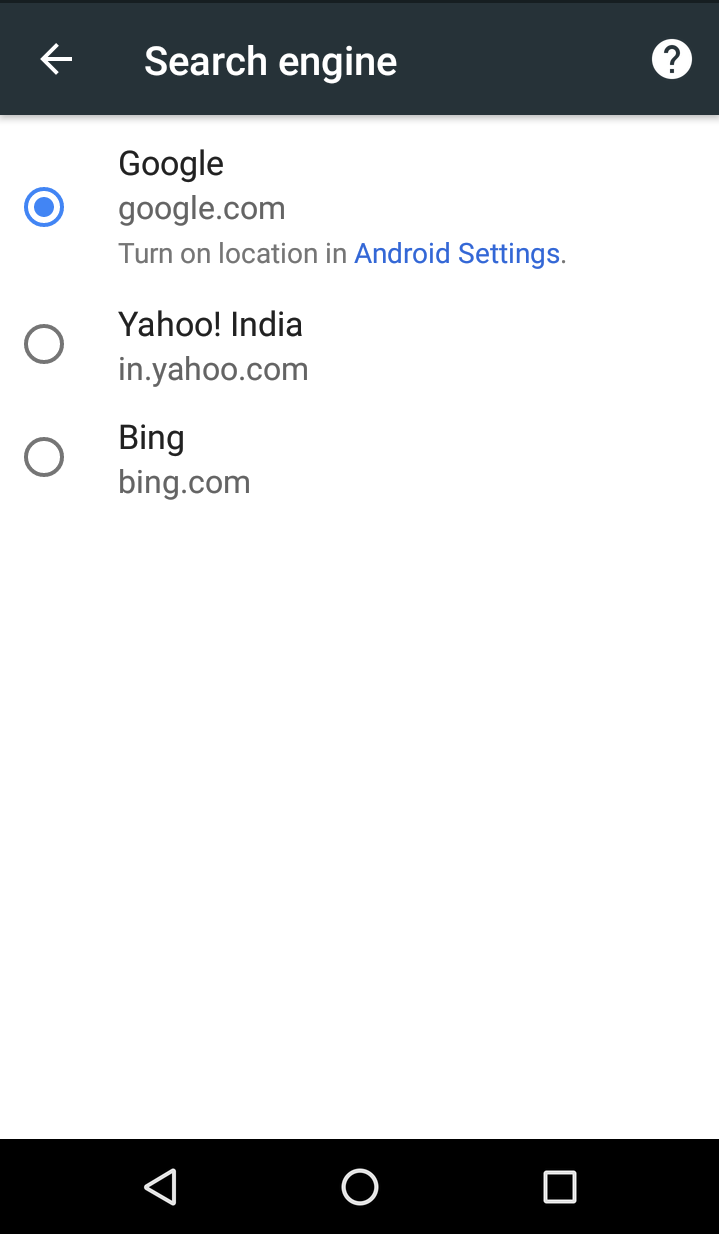The image showcases a user interface screen with a prominent black bar at the top. On the left side of this black bar, there's a white arrow pointing to the left. To the right of the arrow, the text "Search Engine" is displayed. On the far right side of the black bar, there is a white oval shape containing a gray question mark.

Below this, the background transitions to white. On the left side, there are three white circles outlined in black. The top circle is selected, indicated by a blue dot in its center and a blue border. To the right of these circles, text labels indicate search engine options. They are listed as follows: "Google, google.com," accompanied by the instruction "Turn on location in Android settings," with "Android settings" being a clickable blue hyperlink. Below this, "Yahoo India, in.yahoo.com" is listed, and further down, "Bing, bing.com" is displayed.

The rest of the image features a substantial amount of empty white space. At the bottom, another black rectangular shape spans the width of the screen. This bar includes a white triangle pointing left on the left side, a centered circle, and a square with a white border on the right side.